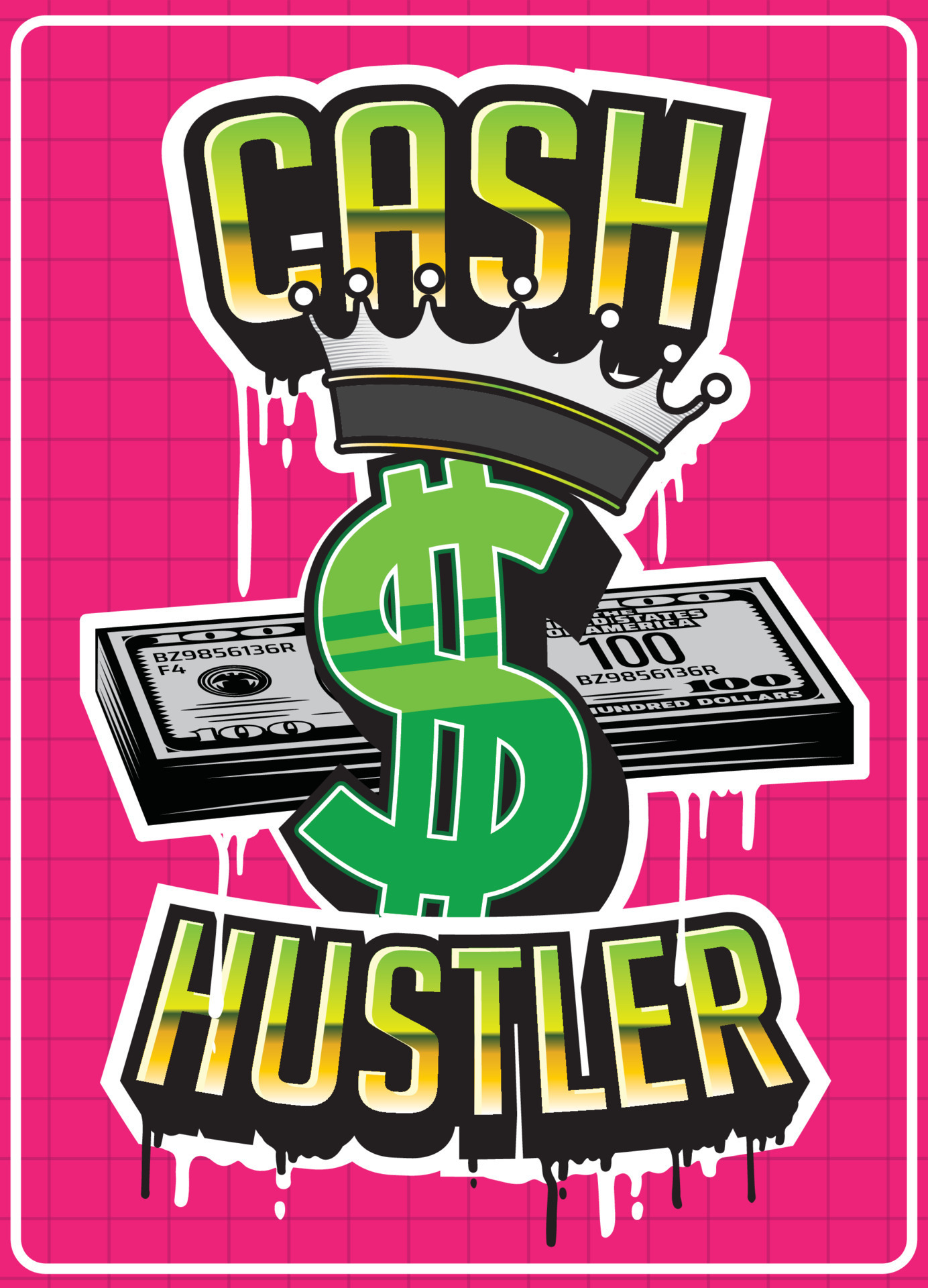The image is a vertically oriented graphic poster with a hot pink background divided into a grid of tiny squares. The centerpiece features the words "Cache Hustler," with "Cache" at the top and "Hustler" at the bottom, written in bold text with a green-to-yellow gradient. A large green dollar sign occupies the center space, adorned with a silver and black crown on top. Behind the dollar sign is a stack of white $100 bills, adding depth to the image. The entire graphic is outlined with a dripping paint effect in black and white, enhancing its stylized, almost spray-painted appearance. The pink background is bordered by a similar hot pink shade, framing the entire composition.